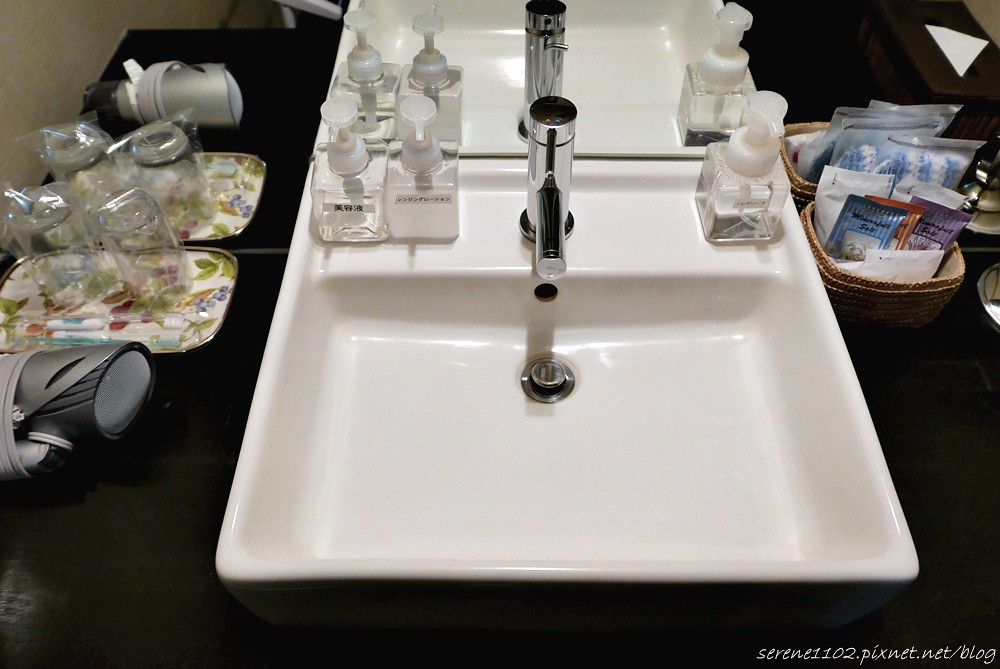This is a photograph of an elegant and minimalist kitchen sink setup. The sink, which is very shallow and square-shaped, appears above the surface of a dark-colored countertop, accentuating its pristine, white cast. A modern chrome faucet stands prominently at the center, with a matching chrome drain situated at the slightly sloped bottom of the sink, ensuring efficient water flow. 

Adjacent to the sink, stylish dispensers with clear bodies and white push tops, likely containing hand lotion and foaming soap, are thoughtfully placed—two on the left and one on the right. The countertop, featuring various odds and ends, complements the sink’s simplistic design.

A large wall mirror situated behind the sink amplifies the space, reflecting the entire setup and adding depth to the scene. In the bottom-right corner of the image, white text reading “serene1102.pixnet.net/blog” is subtly inscribed, marking the source of the photograph. This well-composed image highlights the clean lines and modern aesthetic of the kitchen area.